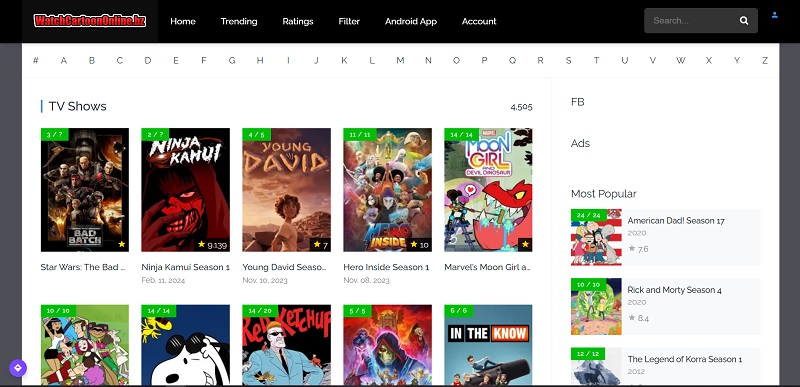In this screenshot from the website WatchCartoonOnline.bz, we can see several interface elements and content listings. The top navigation bar includes tabs for Home, Trending, Ratings, Filter, Android App, and Account, with a search bar and a profile symbol located in the upper right corner. 

The main content area displays a section titled "TV Shows." Directly above this section, there's an alphabet navigation to presumably help users find titles starting with specific letters. The TV shows listed include "Star Wars: The Bad Batch," "Ninja Kamui Season 1," "Young David," "Hero Inside Season 1," "Marvel's Moon Girl and Devil Dinosaur," and an additional partially visible title. Each show on the left side has a green rectangle in the upper left corner indicating viewing progress, such as "3 out of 7" or "4 out of 5" episodes watched.

On the right side of the screenshot, under the heading "Most Popular," another list features "American Dad Season 17," "Rick and Morty Season 4," and "The Legend of Korra Season 1." These popular titles also have green rectangles showing the number of episodes watched.